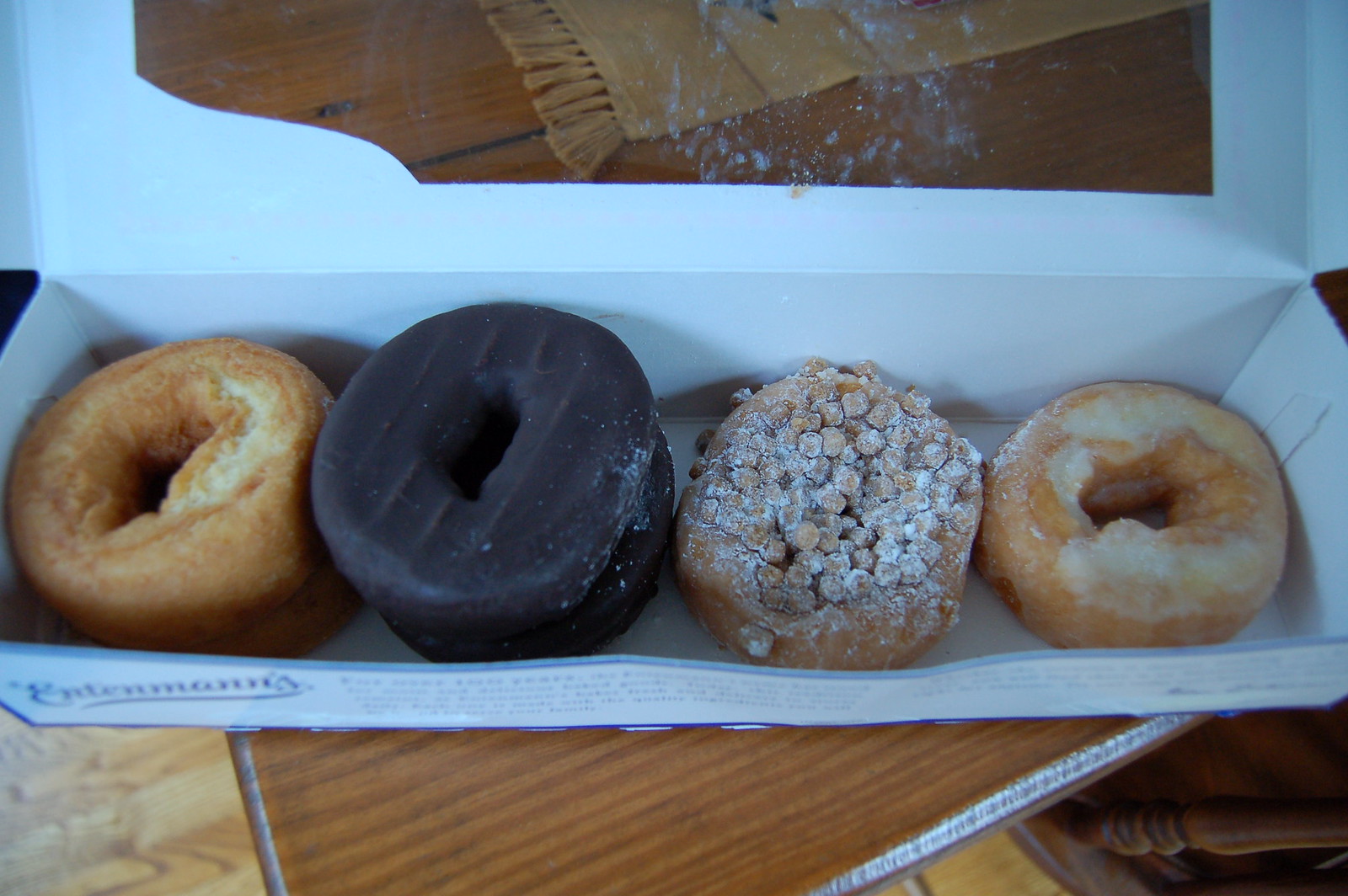In this landscape-oriented photograph, an opened, rectangular white box containing a total of four doughnuts is seen resting on a wooden table. The box features a clear plastic viewing window on the top, and though the company's name in the bottom left-hand corner is out of focus and unreadable, the doughnuts inside are distinct and varied. On the left-hand side are two unglazed, plain cake doughnuts stacked on top of each other. Moving right, the next doughnut is a chocolate-covered doughnut. The third doughnut has a texture reminiscent of a coffee cake, adorned with small bits or possibly nuts. Finally, the fourth doughnut is lightly glazed. The focus of the photograph clearly emphasizes the variety and presentation of these doughnuts within their packaging.